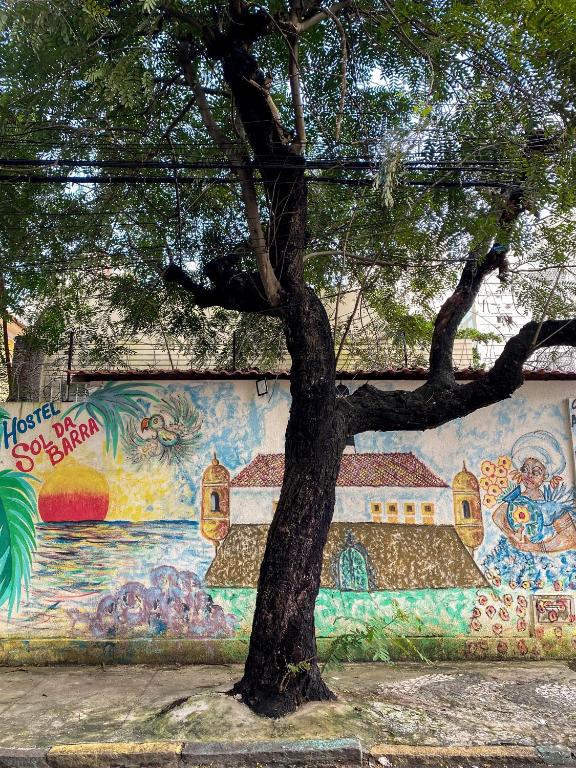This color photograph, taken during daylight, features a tree approximately two feet in diameter growing out of a brown sidewalk in the center of the frame. The tree is surrounded by lush green leaves resembling ferns. In the background, a plaster wall adorned with a vibrant mural captures attention. On the upper left of the mural, bold letters spell out "Hostel Sol de Barra” with "Hostel" in blue and "Sol de Barra" in red. The mural vividly depicts a picturesque scene with a house, a woman wearing a white turban and holding flowers, nearby palm trees, and a sun setting over an ocean horizon. A bird, possibly a parrot, is seen flying across a sunset sky. Electrical wires stretch across the top of the image, and beyond the mural, additional buildings are visible, hinting at an urban environment. The photograph exudes a tropical island atmosphere, evoking a place like Jamaica.